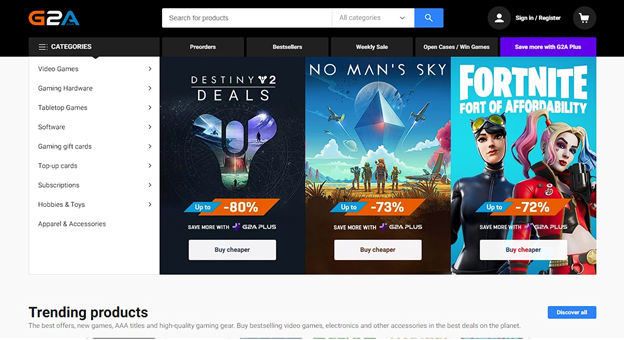In the upper right corner of the webpage, there are options to "Sign In" or "Register," followed by a shopping cart icon. Centrally located, there's a search bar allowing users to search for products, accompanied by a magnifying glass icon for submitting the search query. Adjacent to this is a dropdown menu labeled "All Categories," indicated by a downward-facing arrow. 

On the left-hand side of the page, a vertical navigation menu labeled "G to A" lists various product categories including: Video Games, Gaming Hardware, Tabletop Games, Software, Gaming Gift Cards, Pop-up Cards, Subscriptions, Hobbies and Toys, and Apparel and Accessories. 

The page prominently features games being promoted, starting with "Destiny 2," available for up to 80% off with a clickable "Buy Cheaper" button. Following this is "No Man's Sky," depicted with an image showing jets in the sky and characters with backpacks, offered at up to 73% off, and also includes a "Buy Cheaper" button. Lastly, "Fortnite" is highlighted with a promotion labeled "Fort of Affordability," featuring Harley Quinn and another character wearing yellow glasses perched on her head, available for up to 72% off, along with a final "Buy Cheaper" button.

Below the promotional section, there is a segment titled "Trending Products" with the text in black and a blue rectangle button labeled "Discover All."